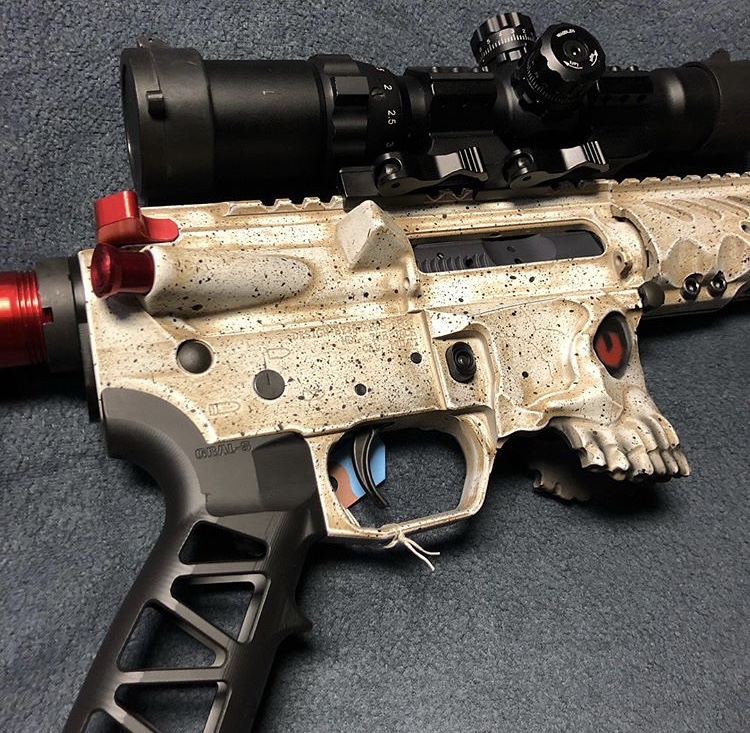The image is a vertical close-up shot of a highly customized rifle resting on a dark gray towel. The rifle, oriented with its barrel pointing towards the right, features a unique and detailed design that blends elements of both real and toy firearms. The handle is black with cutout triangles, giving it a tactical appearance. The main body of the rifle has a light brown to off-white color with a speckled black pattern, evoking a skull-like aesthetic. 

The stock and other parts of the gun display a skull design, complete with detailed red highlights for eyes and teeth, enhancing its menacing look. The trigger is predominantly black, and nearby, there are several red projections and a circular red object emerging from the gun. 

Above the main body, the rifle is equipped with a large, functional-looking black scope. The scope has a tube-like appearance with a matte finish and is fitted with dials for sight adjustments, featuring visible numbers like 2 and 2.5. The intricate design suggests it could be used for precise targeting, reinforcing the weapon's elaborate and possibly decorative nature.